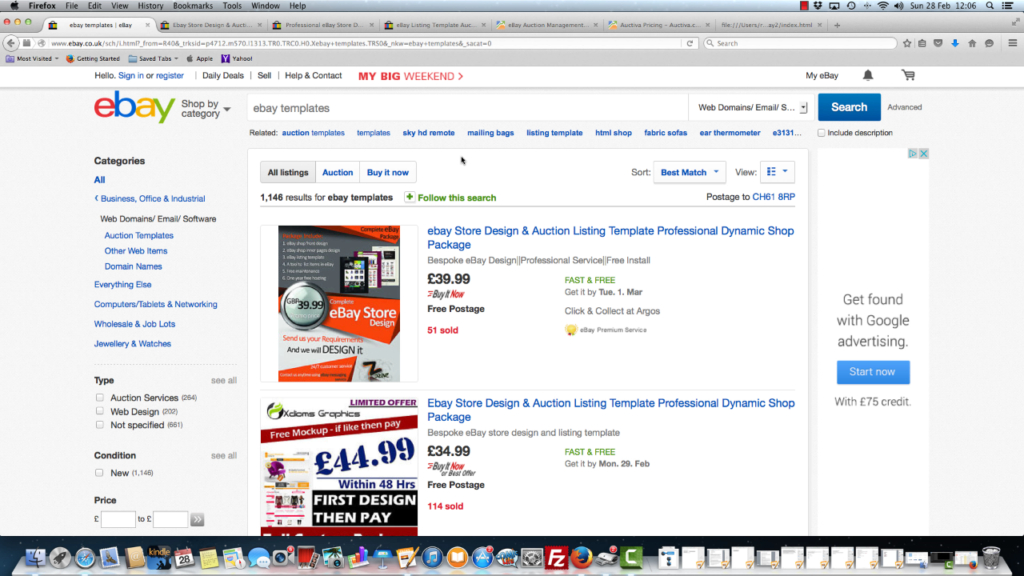This screenshot captures a screen grab from an Apple computer displaying a web browser with multiple open tabs. The focus is on the first tab, showcasing the eBay website. At the top of the screenshot, the Apple navigation bar is visible, featuring the Apple logo on the top left corner, alongside various menu options such as File, Edit, and View. On the right side of the navigation bar, the date, time, and other Apple system icons are present.

Below the Apple navigation bar, the browser’s address bar shows that the current website being viewed is eBay. The left sidebar of the eBay site, set against a pale grey background, has a "Shop by category" section listing various categories. The main content area, on a white background, prominently displays two eBay store design and auction listing template packages. The first package is priced at £39.99, while the second one is listed at £34.99.

On the right side of the webpage, there is a white space allocated for advertisements, currently showing a promo for Google advertising, offering a £75 credit to "Start now." 

At the bottom of the screenshot, the macOS taskbar is visible, displaying icons for different programs and open documents, facilitating quick access to various applications.